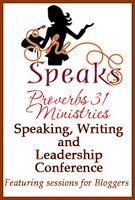The image is a detailed advertisement for the "She Speaks" conference organized by Proverbs 31 Ministries, focused on speaking, writing, and leadership, with special sessions for bloggers. Dominating the image is a poster entirely filling the rectangular frame with a thin, light brown border. At the top of the poster is a central, solid black silhouette of a woman in a side profile, her long hair flowing and one hand gesturing while she speaks into a microphone. Below the illustration is the text "She Speaks" in large, ornate letters with a swirly 'E'. The subsequent lines of text state "Proverbs 31 Ministries, Speaking, Writing, and Leadership Conference," followed by a smaller, italicized line that reads, "featuring sessions for bloggers." The lettering colors vary, including black, brown, maroon, and pink, contributing to the sophisticated and inviting design of the poster promoting the upcoming religious event.